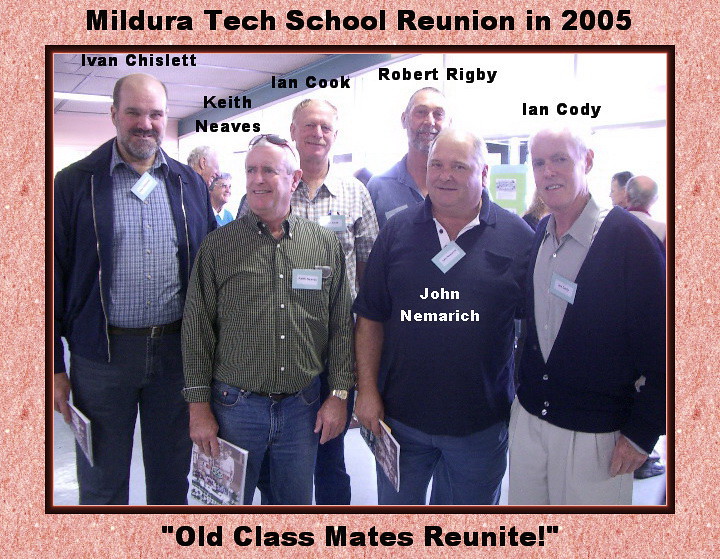This image captures a rectangular photograph against a subtly textured pink background, framed by a brown border. The border features black text at the top reading "Mildura Tech School Reunion in 2005" and along the bottom, “Old Classmates Reunite.” The photograph showcases six elderly men standing in a room, seemingly at ease while posing for the picture. Their names are labeled above their heads, proceeding left to right: Ivan Chislett, a tall, bald man in blue; Keith Neves, who has gray hair and is dressed in a green shirt and blue jeans; Ian Cook, positioned behind in the row; Robert Rigby, whose name is also written on his stomach area; Joan Nemerick, a shorter man in front of Robert Rigby, wearing a blue polo shirt and jeans; and Ian Cody on the far right. The backdrop reveals parts of the room’s interior, including visible windows and figures, hinting at a lively reunion atmosphere among old classmates.